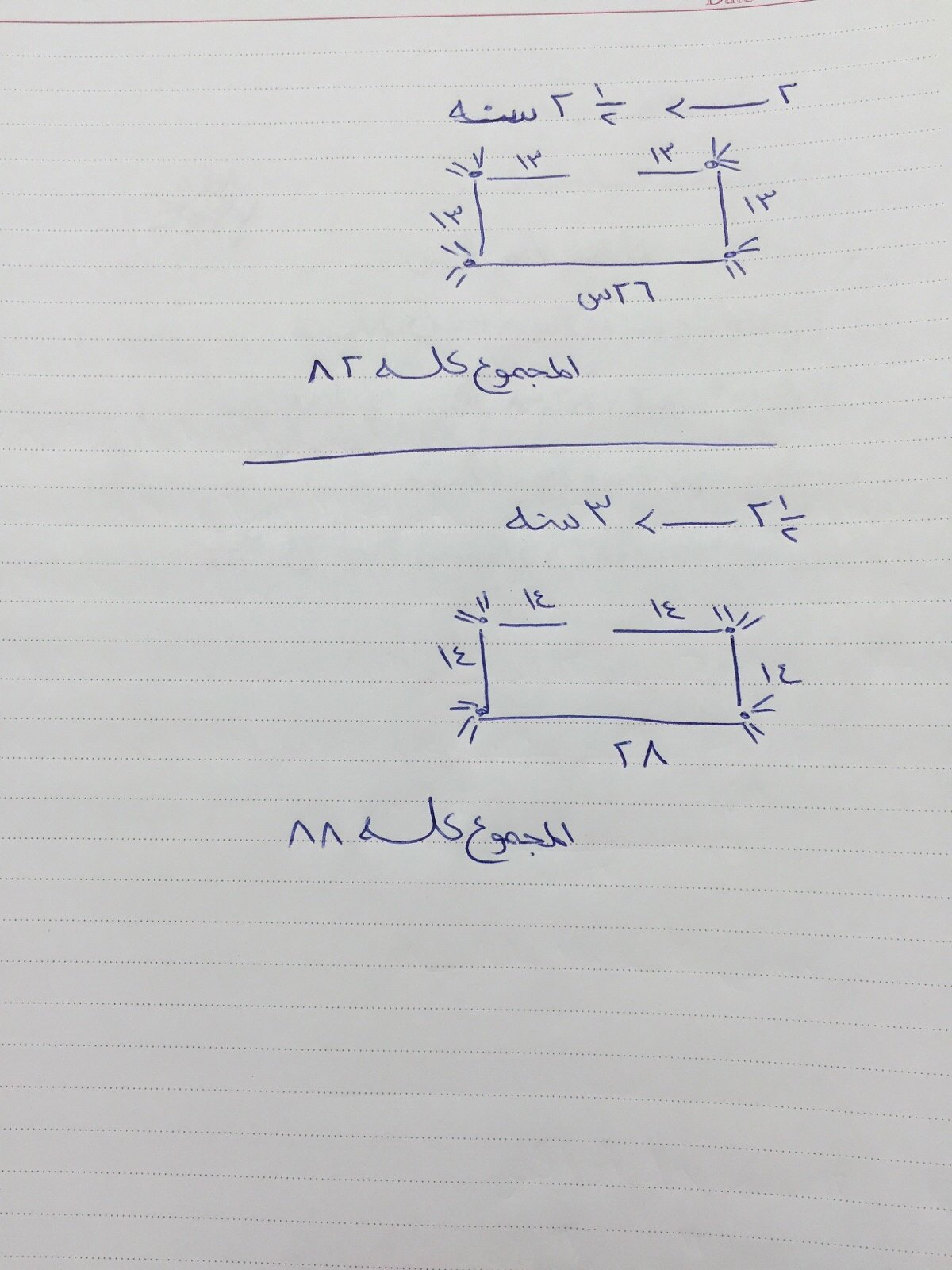A white piece of lined notebook paper is covered with intricate blue ink drawings that appear to be mathematical equations. At the top of the paper is a rectangular shape, but the top line of the rectangle is incomplete, leaving a small gap in the middle. Surrounding the corners and sides of this rectangle are pairs of short dashes, giving it a segmented appearance. Within the rectangle, there are symbols resembling fractions, with a numerator that looks like the number "1" and a denominator that appears to be a backward "R". 

Beneath this shape is a statement written in what looks to be a non-English script. One character resembles an uppercase "A" without the middle line, another looks like a backward "R", and yet another similar to a lowercase "a" with an extended tail. 

Following this, there is a horizontal blue line and another sequence of complex mathematical symbols. Further down the page, there is another rectangular figure with an incomplete top line, similar to the first, featuring the same segmented dashes at the corners. Surrounding this figure, there are what seem to be Latin letters alongside another array of mathematical notations. At the bottom of the page is yet another set of symbols that do not resemble English or standard numerical characters, appearing more like Greek or Latin script.

This detailed and highly mathematical document suggests the use of specialized notation, possibly for advanced mathematical or linguistic problems.